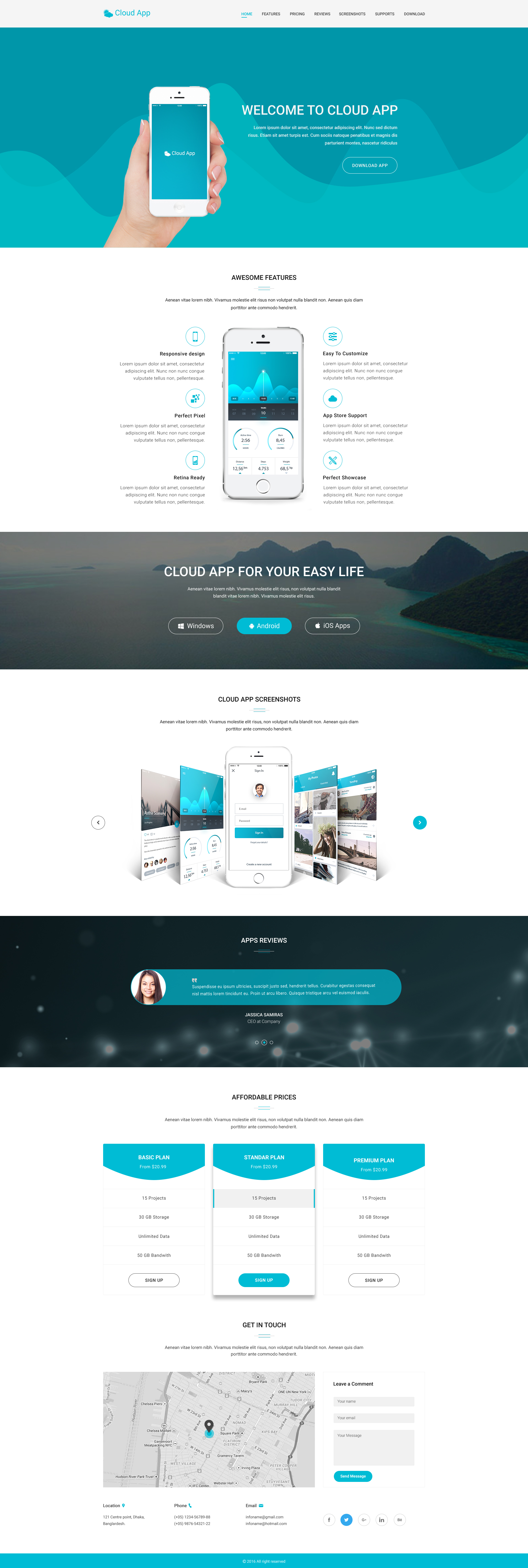This portrait-oriented screenshot intricately showcases a promotional page for the "Cloud App". At the very top, from the upper left to the upper right corner, the words "Cloud App" are prominently displayed, while smaller text is not discernible. Beneath, a teal abstract design forms the background, setting a dynamic tone. 

On the left side of the image, a light-skinned hand with visible fingernails delicately holds a digital image of a white cell phone. Centrally placed, the name "Cloud App" is reaffirmed, and the right column features a welcoming message, "Welcome to Cloud App," accompanied by a clear "Download App" button.

This comprehensive page is dedicated to advertising the "Cloud App" and introduces its "Awesome Features" right below. Here again, another cell phone image is displayed, possibly showing a video to highlight the app’s functionalities. 

The following section portrays a dark scenic backdrop of an ocean against mountains, with the phrase "Cloud App for your easy life" boldly centered. Three buttons below this header indicate compatibility with Windows, Android, and iOS apps, with the Android button highlighted in light blue, suggesting it is selected. 

Further down, the screenshot mentions "Cloud App Screenshots" and offers navigation with teal right and left arrows to browse through different screenshots. 

The subsequent sections feature "App Reviews" followed by information on "Affordable Prices," enriched with numerous forms for user interaction and feedback. Concluding the informative journey is a map, providing visual context or possibly user locations.

This image captures the essence and functionality of the Cloud App, blending visual appeal with detailed technical information.